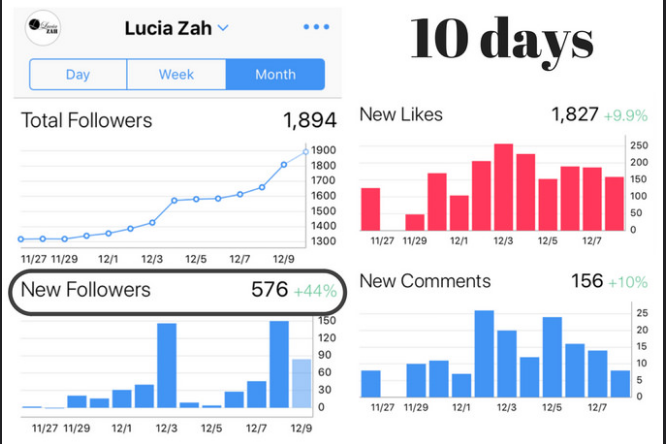The image displays a detailed analytics dashboard for user Lucia Zas, organized into four stacked quadrants. At the top, it features the username "Lucia Zas" in black text, along with clickable viewing options: day, week, and month. The graphs showcase different metrics over a date range from 11/27 to 12/09. 

In the upper left quadrant, a line graph titled "Total Followers" displays a total of 1,894 followers, indicating a 13.8% increase. Below it, a bar chart labeled "New Followers" shows 576 new followers, reflecting a 44% rise. 

In the right column, the top quadrant contains a red bar chart labeled "New Likes," with a total of 1,827 likes and a 9.9% increase. Below it, a blue bar chart labeled "New Comments" indicates 156 new comments, marking a 10% increase.

Overall, the dashboard provides a clear visual representation of user engagement over the past 10 days, with both line and bar charts highlighting key performance metrics.